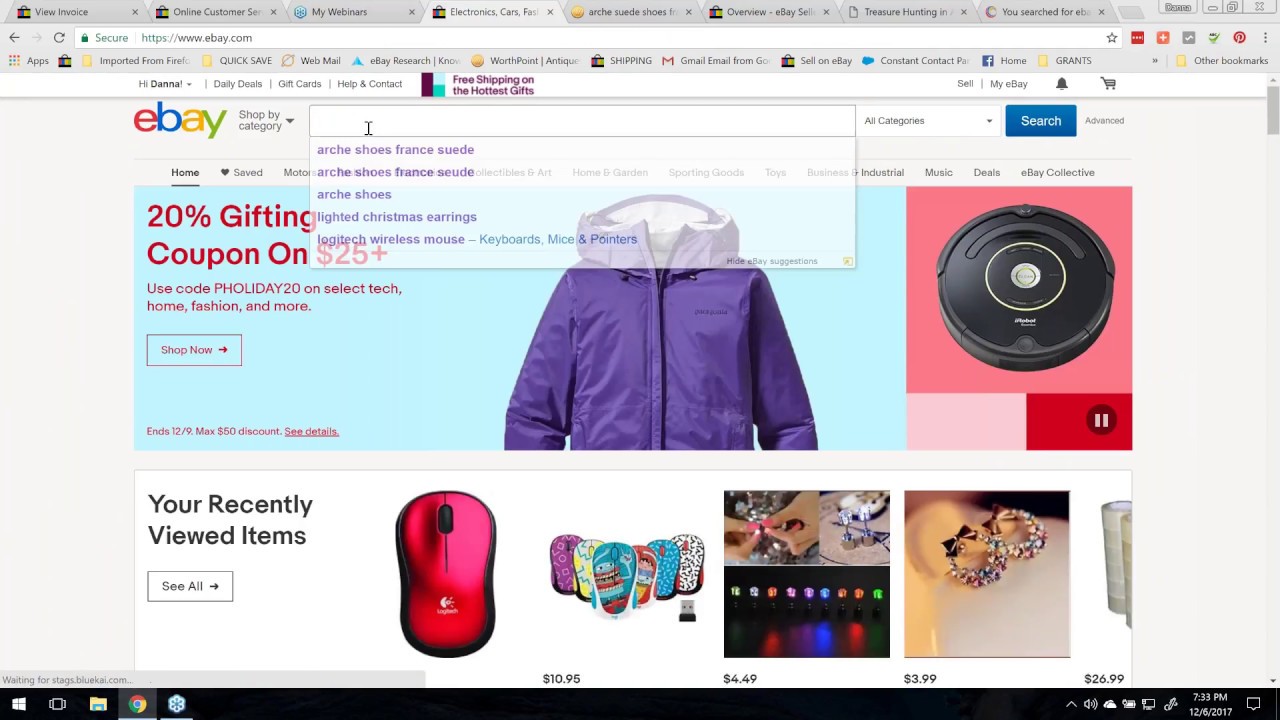Displayed on the computer screen is a web browser with the eBay homepage open. The top of the screen shows a row of tabs, around ten visible, indicating multiple sites and pages the user has been visiting. Additional tabs are grouped within an aggregator, suggesting extensive web browsing activity. The browser’s search bar reveals the user navigated to ebay.com, leading to the current view of the eBay website.

Below the search bar are familiar browser elements: navigation buttons, bookmark shortcuts, and various app icons installed on the computer. The eBay site itself features the iconic logo, with a red 'e', blue 'b', yellow 'a', and green 'y', representing its brand. The homepage prominently announces a holiday sale offering a 20% discount on selected items.

Highlighted in the center of the page is an image of a floor vacuum robot, showcasing one of the items on sale. Additionally, search results for "arch shoes" are displayed, indicating the user's recent query on eBay. The screen provides a typical, yet comprehensive glimpse into the user's online shopping and browsing activities.